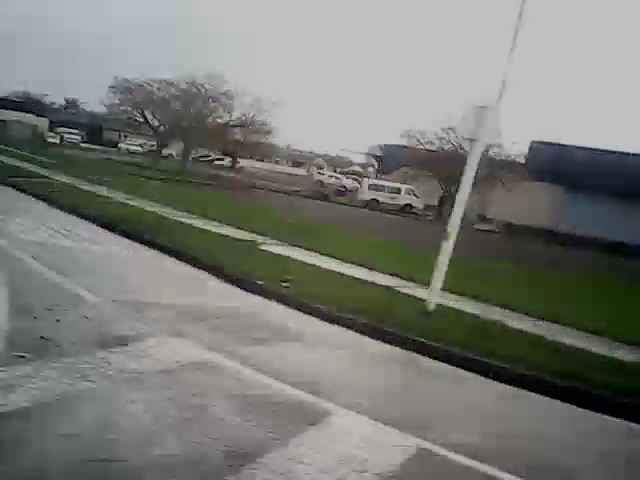The image appears to be a dash cam screenshot taken outdoors during the late afternoon. The top half of the image shows a hazy, gray sky with some clouds, indicative of an overcast day. Below the sky, several leafless, brown trees are visible around a parking lot light structure, with three trees on the left side and one on the middle right. The parking lot is filled with various vehicles, including a white van, an SUV, and a sedan. The pavement of the parking lot is gray cement. In the bottom half of the image, a grassy area flanks a sidewalk, which features a large white lamp post. Further detail includes a street with white paint markings, indicating it's a road with delineated lanes. The overall impression is that the scene captures a commercial area with buildings, parking lots, and minimal greenery.